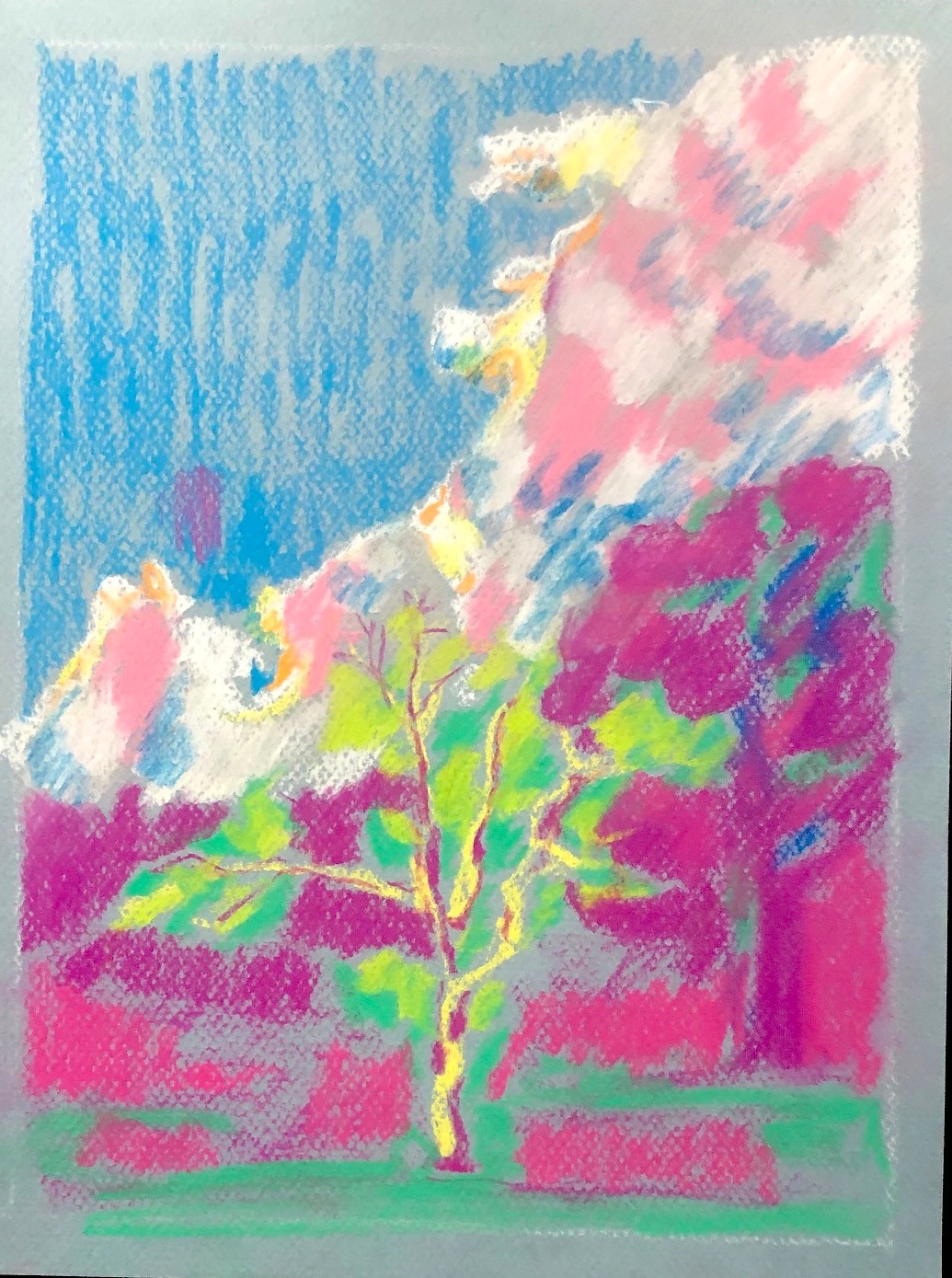The image is a detailed artwork, likely created with oil pastels on textured gray paper, depicting a vibrant and colorful landscape. The central feature is a tree adorned with leaves in various shades—red, yellow, and green. Surrounding the tree, angled red and blue striations add texture to the scene. In the background, a second tree, highlighted in red with blue accents or perhaps a blue backdrop, creates a dynamic contrast. The background also suggests the presence of a mountainous landscape with gray and white, possibly indicating snow-capped peaks. The sky is rendered in blue, albeit with a somewhat scribbled technique. Despite the youthful execution, the composition encapsulates a lively nature scene with additional elements like branches and leaves, all enclosed within a frame, underscoring its presentation as a standalone piece of framed art.